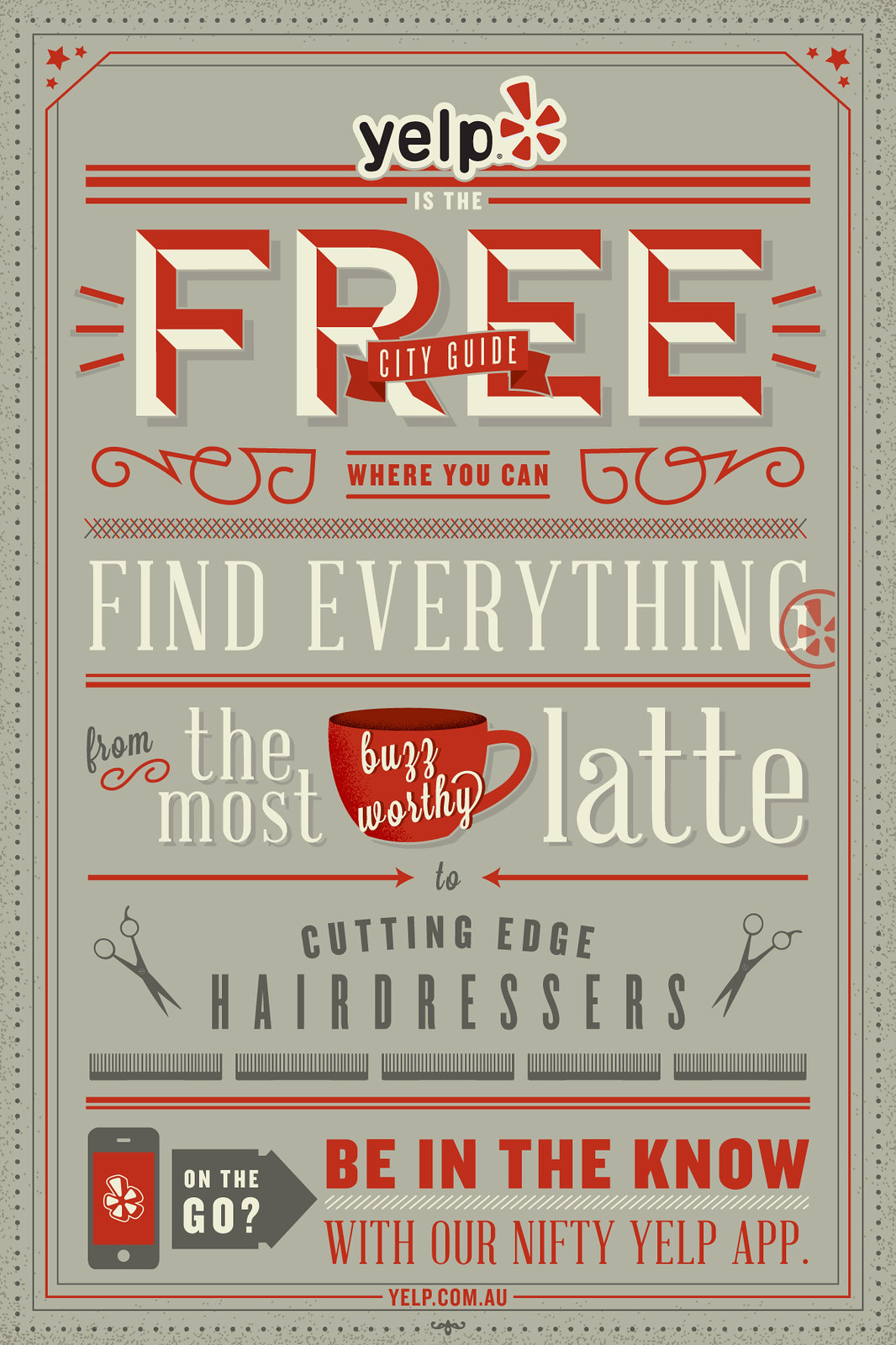The Yelp advertisement features a detailed and vibrant design. It has a light gray background with several borders: a dotted blue line, a solid blue line, a red line with stars in the corners, and another solid blue line. At the center, the bold name "Yelp" is accompanied by their signature asterisk logo and the tagline "Yelp is the free city guide where you can find everything." The text prominently highlights in large red and white letters the word "FREE." Below this, the text elaborates, "From the most buzzworthy latte," with an illustration of a red cup behind the phrase, and "To cutting-edge hairdressers," featuring a pair of gray scissors and a row of combs. The advertisement concludes with, "On the go, be in the know with our nifty Yelp app," and showcases an image of a phone displaying the Yelp app. The majority of the text is in red or white, enhancing readability against the gray backdrop. The ad effectively emphasizes the comprehensive and practical uses of Yelp for various needs and services.